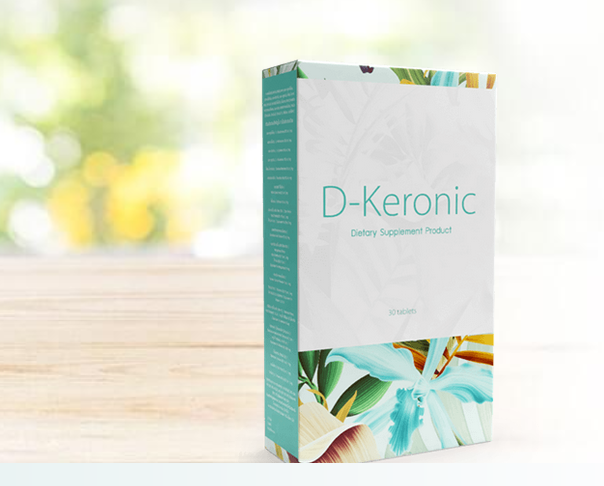The photograph captures an image of a teal, rectangular box prominently set in the foreground. The box showcases a vivid floral design featuring blue, red, and yellow flowers intertwined with green leaves. The front of the box is dominated by a white label positioned centrally that bears the text "D Keronic" in teal letters, followed by the words "dietary supplement product" in smaller letters, and near the bottom, "30 tablets." The sides of the box also feature teal labels with white text, though the lettering is too small to discern. The box is angled and rests upon a faded, slightly stained, light wooden table. In the backdrop, the scene is blurry and washed-out, hinting at greenery and possibly yellow flowers, suggesting they might be arranged in a basket.